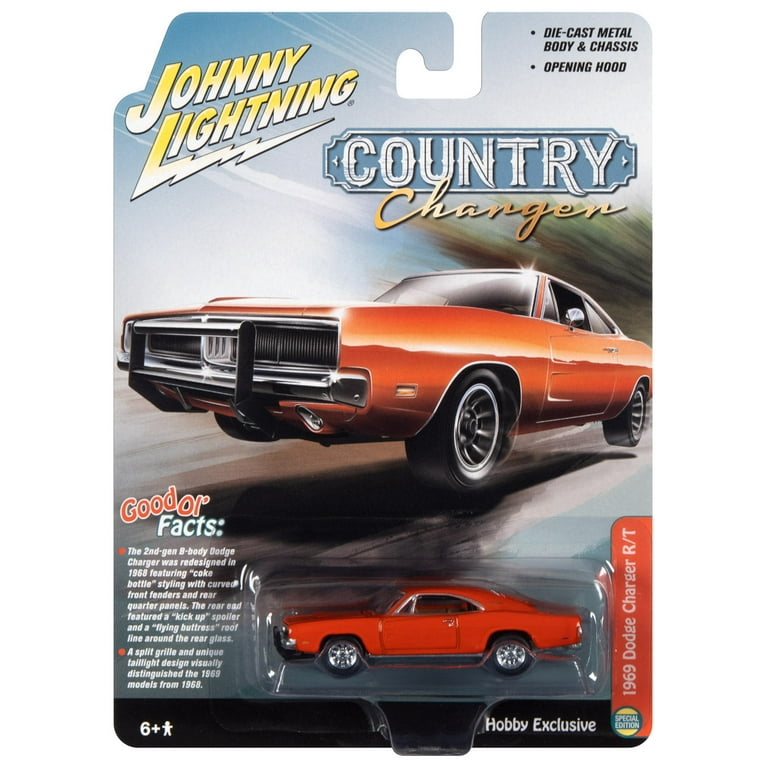This image displays a Johnny Lightning Country Charger toy car, mimicking the style of Hot Wheels, securely encased in plastic and attached to a printed cardboard backing. The main focus is an orange 1969 Dodge Charger RT, prominently indicated as a special edition with a red label. Positioned at the top left corner, the Johnny Lightning logo is visible with a trademark symbol. At the top right, the package highlights the toy's features: a die-cast metal body and chassis with an opening hood. The header of the package has a hook slot for store display.

The center of the card features an illustration of the Dodge Charger, depicted with a blurred background to suggest speed. Underneath, a section titled "Good or Facts" provides detailed information about the car's design evolution, including the distinctive coke-bottle styling from 1968, updates to the curved front fenders, rear quarter panels, kick-up spoiler, flying buttress roofline, split grill, and unique tail light design which differentiate the 1969 model from its predecessor. At the bottom left of the card, a small black-bordered box indicates that the toy is suitable for ages 6 and up. On the right, a label specifies this as a "Hobby Exclusive."